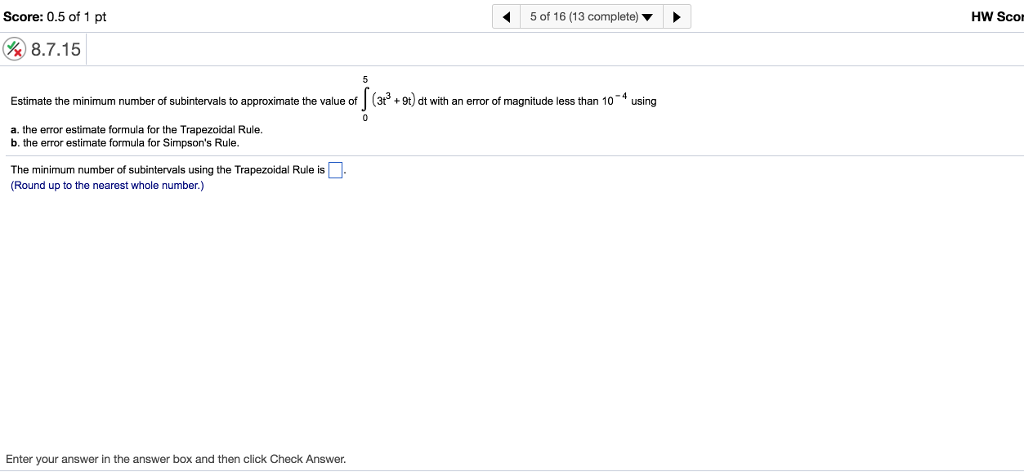Screenshot of a MyMathLab testing page displaying results for a college-level math question. The screenshot shows the interface of an online math assessment, commonly utilized in college courses. At the top left corner, it indicates a score of 0.5 out of 1 point for Question 5 of 16. The progress tracker reveals that 13 questions have been completed out of the total 16. 

The main content of the page reads:

**Estimate the minimum number of subintervals to approximate the value of** 

\[ \int_{0}^{5} (3t^3 + 9t) \, dt \]

**with an error of magnitude less than** 

\[ 10^{-4} \] 

**using:** 
- **(A) the error estimate formula for the trapezoidal rule**
- **(B) the error estimate formula for Simpson's rule**

Below the instructions, it asks for the minimum number of subintervals needed using the trapezoidal rule, which is currently unanswered. Despite the lack of visible answers on the page, the score shows that half a point was awarded for this question.